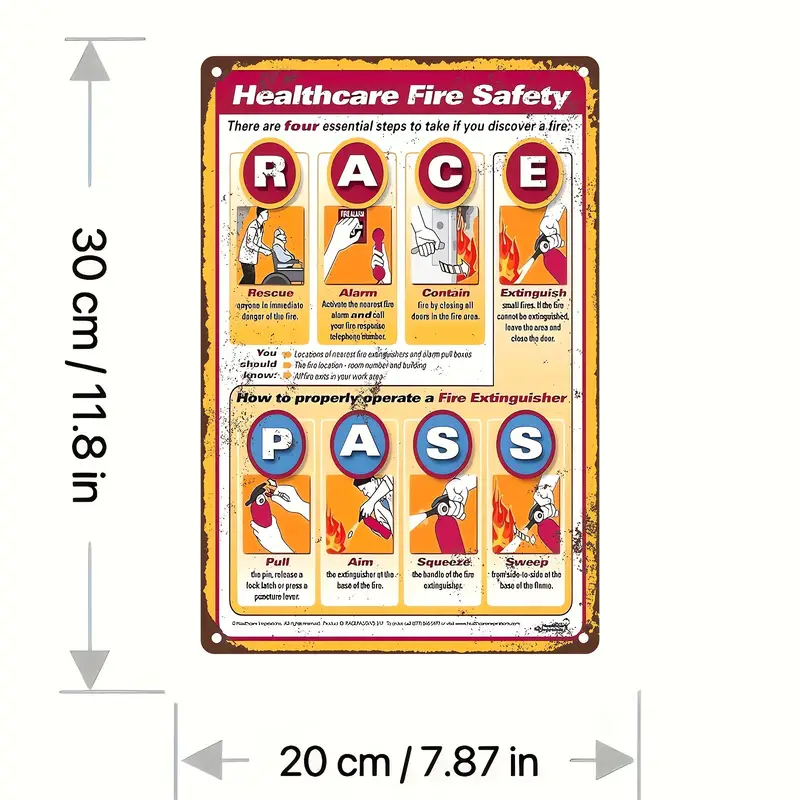The image features a very old-fashioned metal plaque focused on health care fire safety, with detailed instructions. The plaque is clearly metal, indicated by four mounting holes at each corner, and shows signs of age with chipping paint and visible rust. At the top of the plaque, vibrant white letters on a raspberry-colored background spell out "Health Care Fire Safety." Below this title, prominently displayed in red oval frames, are the letters "RACE," an acronym for the four essential steps to take in case of a fire: Rescue, Alarm, Contain, and Extinguish. Additionally, the bottom section of the plaque details the acronym "PASS" for operating a fire extinguisher—Pull, Aim, Squeeze, and Sweep—all illustrated with specific graphic depictions. The plaque includes measurements on the sides and bottom, indicating its suitability for placement in commercial spaces such as kitchens or factories where quick access to fire safety instructions is crucial.